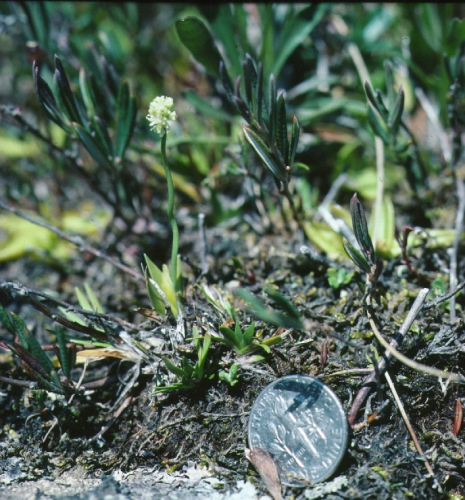This is an extreme close-up photo of the ground, showing a small mound of earth with diverse details. The central focus is a dime, resting on its side and showing its backside, which provides a clear perspective of the scene's scale. Surrounding the dime, tiny blades of grass and small sticks are sprouting from the dirt, creating a textured foreground. Prominently visible is a very small plant with a stem only an inch or two tall. At the top of this stem, a tiny white flower is just beginning to bloom. The background is blurred, emphasizing the detailed features in the foreground, and hints of green suggest a sunny day. This tiny ecosystem of dirt, emerging grass, and the budding flower captures a vivid and intimate moment of nature's growth.